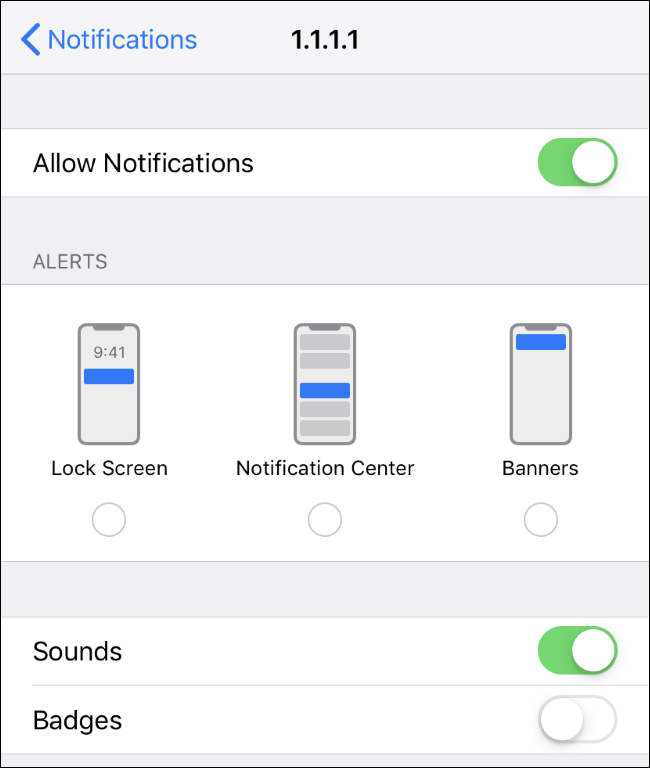This image shows a detailed screenshot of an admin panel for managing notifications on a mobile phone. At the top of the screenshot, there is a back arrow on the left and the word "Notifications" displayed in blue text. Below this, the text "1.1.1.1" is visible followed by a light gray bar. Underneath the bar, there is a white section with the text "Allow Notifications," which is currently enabled, as indicated by a green sliding button.

Further down, there is a gray panel labeled "Alerts." Below this panel, three phone mockups are displayed side by side. 

- The first mockup on the left is labeled "Lock Screen," showing the date and a blue notification panel.
- The middle mockup is labeled "Notification Center," highlighting a blue notification approximately halfway down the list, flanked by two gray notifications above and two below.
- The third mockup on the right is labeled "Banners," displaying a blue notification rectangle near the top.

Below these mockups, there are circles under each notification option, indicating the option to select one. There is a blank field beneath these circles.

Further down, there are options for "Sounds" and "Badges." The "Sounds" option is currently enabled, as shown by the on position of the slider, while "Badges" is off.

The entire screenshot is outlined by a thin, single black pixel line in a rectangle with sharp corners.